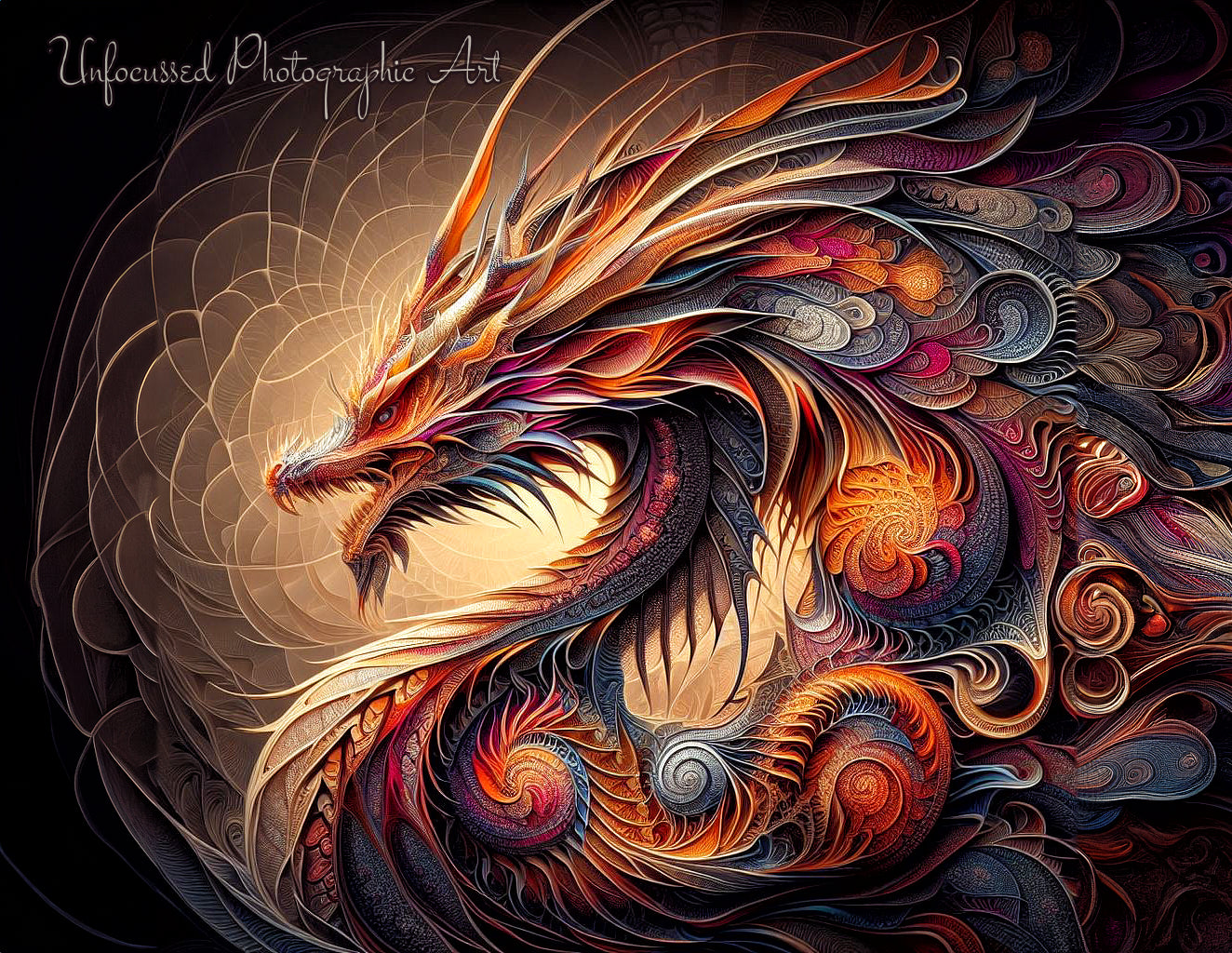This vibrant digital art image showcases an intricately detailed, Asian-style dragon rendered in high definition. The dragon, depicted from a side view, features a dynamic array of colors including prominent shades of pink, red, yellow, blue, and particularly orange, which highlights its scales and teeth. The dragon's design boasts curvy, flowing lines, with hair-like elements and swirling patterns adding to its majestic appearance. The background is predominantly yellow with subtle brown shapes, and blues and grays on the far right, enhancing the depth of the scene. Text in the upper left corner reads "unfocused photographic art" in gray, adding a mysterious touch to the overall composition.